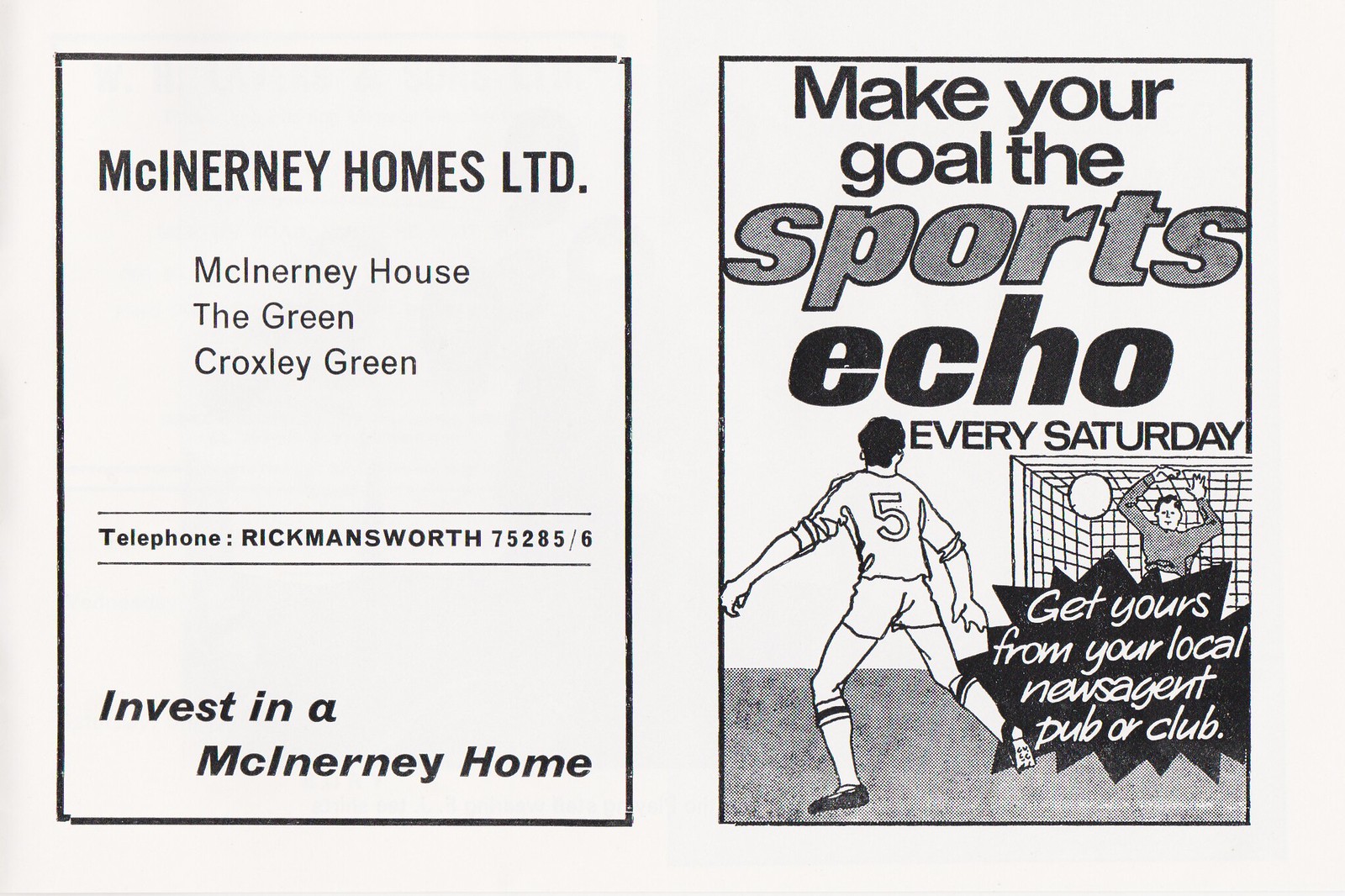This image is designed to resemble an open book or a pamphlet, presenting two distinct advertisements on adjacent pages. On the left page, there's a black and white advertisement for McKearney Homes Limited, located at McKearney House, The Green, Croxley Green, Rickmansworth. The text encourages viewers to "invest in a McKearney home." 

The right page showcases a promotion for "Make Your Goals Sports Echo," emphasizing its availability every Saturday and advising readers to get their copy from their local newsagent, pub, or club. This section includes a detailed drawing featuring two people playing soccer. The player with black hair, donning a number five uniform, is seen kicking the ball towards the goal. The goalkeeper, arms raised in an attempt to block the incoming shot, adds a dynamic element to the scene, which is set against a white background with a grassy field. Both players are equipped with socks and cleats, underscoring the sporty theme of the advertisement. The overall color scheme is black and white with some text appearing in a pinkish shade.